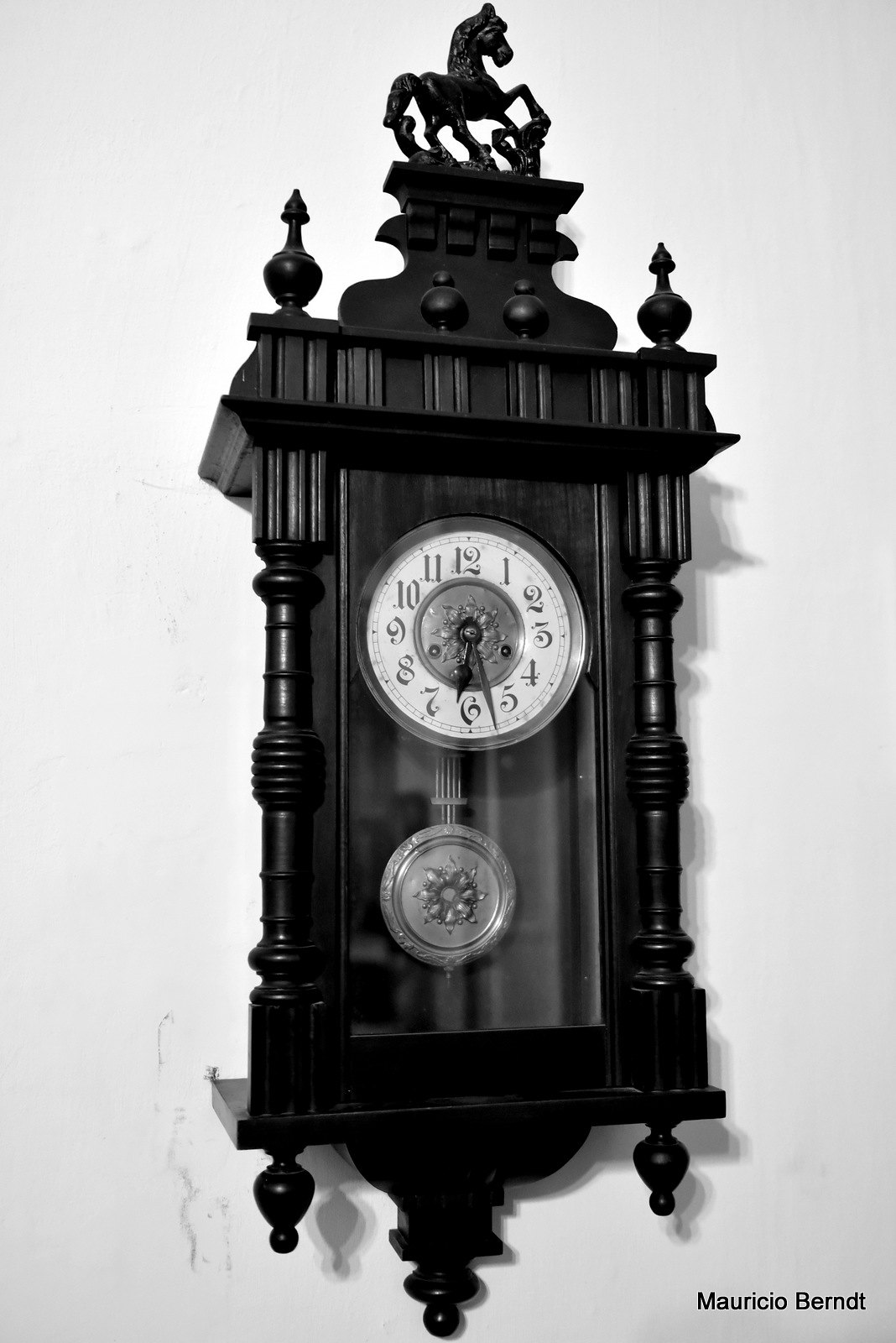This meticulously detailed black and white photograph captures a beautifully ornate wall-mounted clock. Encased in what appears to be a finely-crafted wooden structure, the clock features an intricate decorative outer shell. At the pinnacle of this elegant timepiece sits a sculpted horse, which adds a touch of regal charm. Below the horse, the body of the clock includes rounded sections, framing it with a sense of harmony and balance. The sides are accentuated with small wooden pillars that enhance its classical aesthetic.

The clock face itself is a captivating focal point, boasting a white background with an intricately designed inner section. The numerals, though slightly unconventional in font, remain clear and easily readable, contributing to the clock's unique character. Directly beneath the clock face, a graceful pendulum is visible, swinging with timeless rhythm. Both the clock face and the pendulum are encased behind a pane of glass, offering a subtle gleam that complements the overall vintage elegance of this distinguished timepiece.